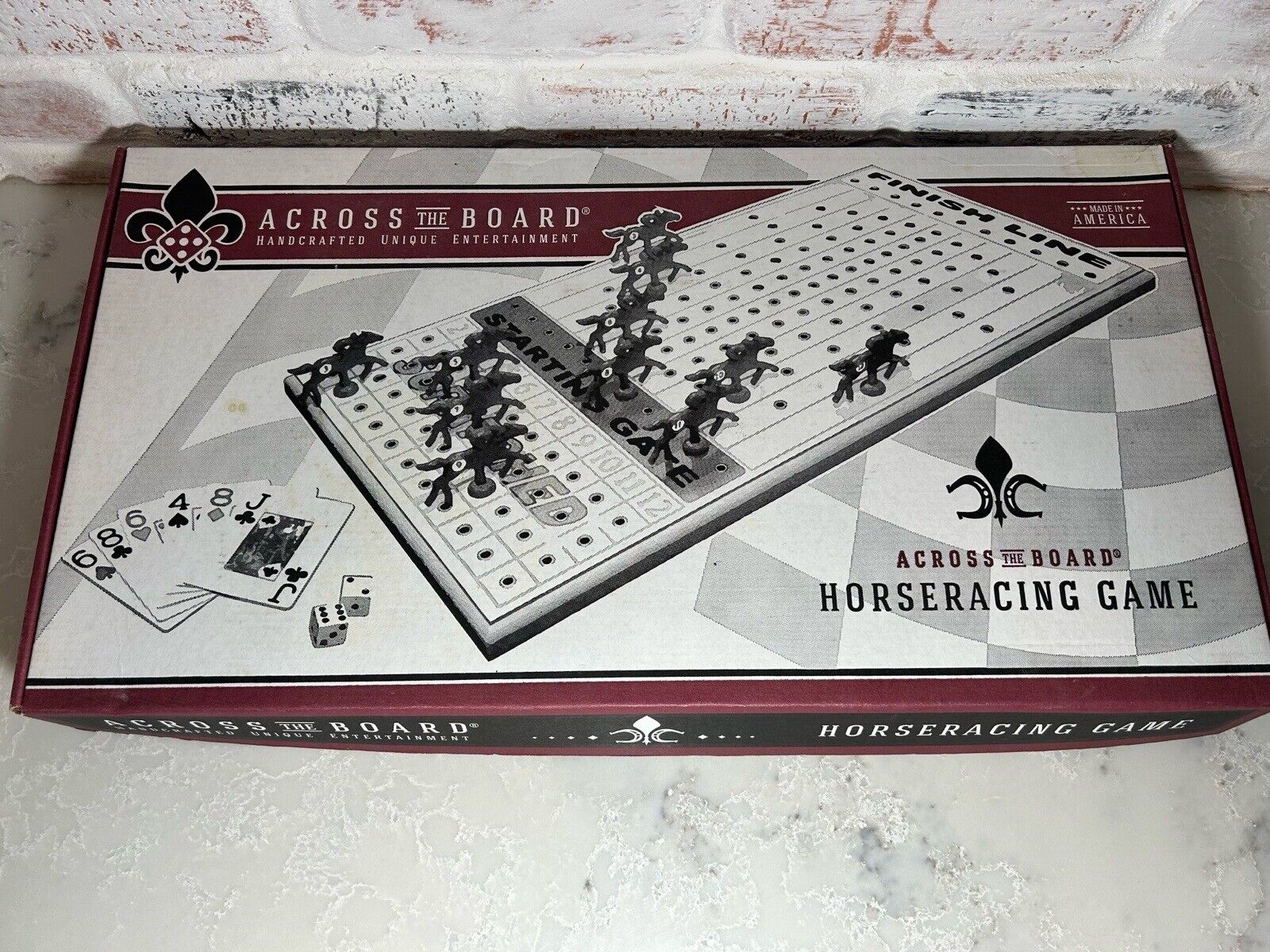The image depicts a detailed board game called "Across the Board: Horse Racing Game," set against a backdrop of a painted-over brick wall, featuring white paint over blue. The board game is positioned on a white marble floor with black spots. 

At the upper left corner of the game, it says "Across the Board, Handcrafted Unique Entertainment" with the image of a dice showing the number five in front of a black Fleur-de-lis. The upper right corner of the game mentions "Made in America." The main playing area of the game features a black, white, and gray board, prominently displaying the "Starting Gate" and a series of horses, indicating the beginning of the race. 

In the lower left corner, a collection of playing cards (6-8-6-4-8 Jack) and a set of dice (showing six and two) are visible. Additionally, it features a red stripe that intersects the board and displays the game's name, "Across the Board." The lower right corner highlights two horseshoes alongside the name "Across the Board: Horse Racing Game." The board's design suggests that players move horses on pegs from the left side, the "starting gate," to the right side, the "finish line."